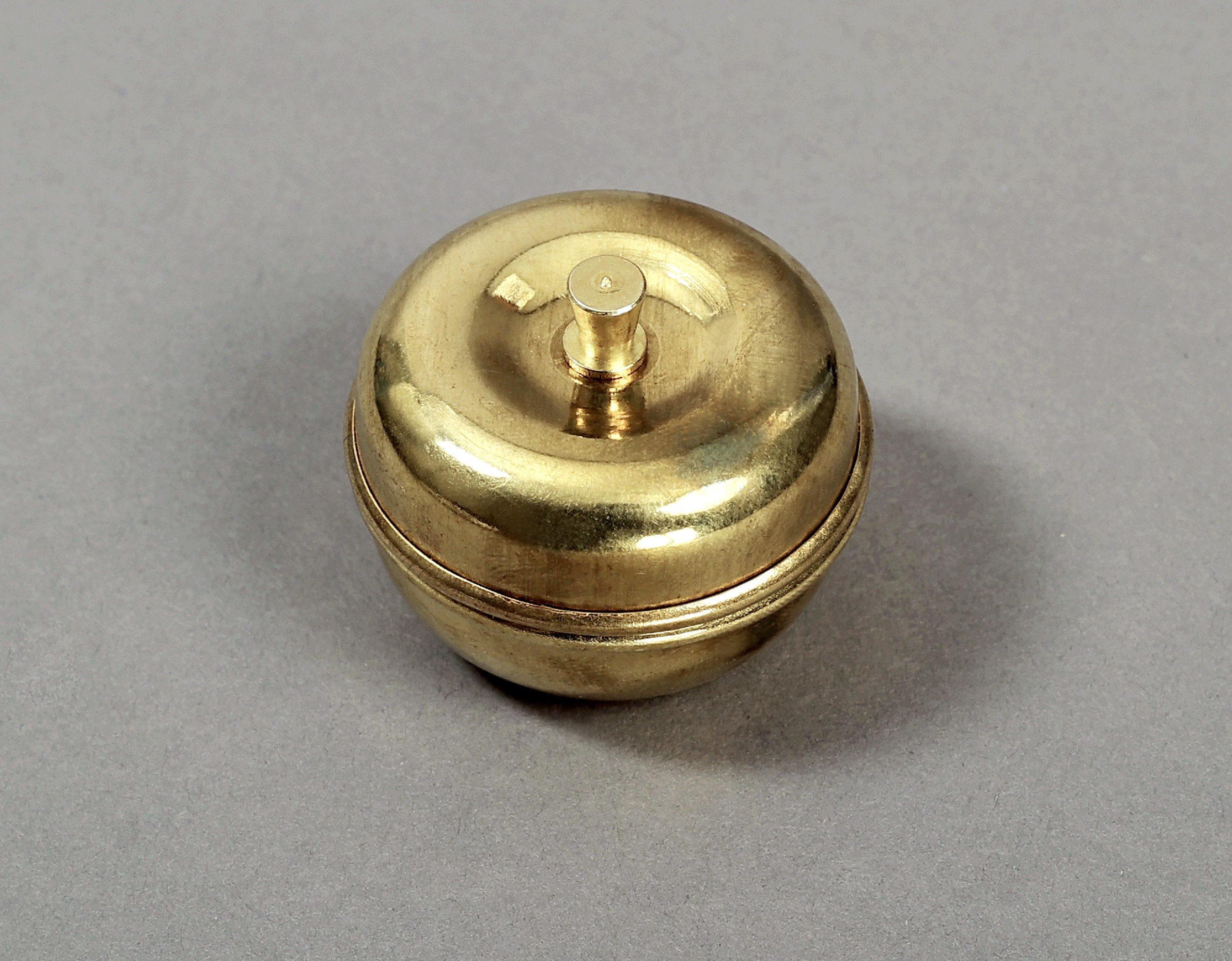The image displays a bronze ornament, predominantly gold in color, resting on a uniform gray surface. The ornament is shaped somewhat like a spherical object with a flat top and bottom, resembling an apple or a doorbell. At the top, there is a distinctive knob or handle, which is narrower in the middle and widens into a flat, circular top, reminiscent of a small top hat. This knob sits in a dimple at the upper half of the ornament. The object is divided horizontally through the middle, creating two hemispheres, and a shadow extends to the right side due to a light source above. Various reflections from the light illuminate different parts of the ornament, particularly highlighting its golden hue. On closer inspection, the design suggests it could serve as a jewelry holder or a decorative antique piece.